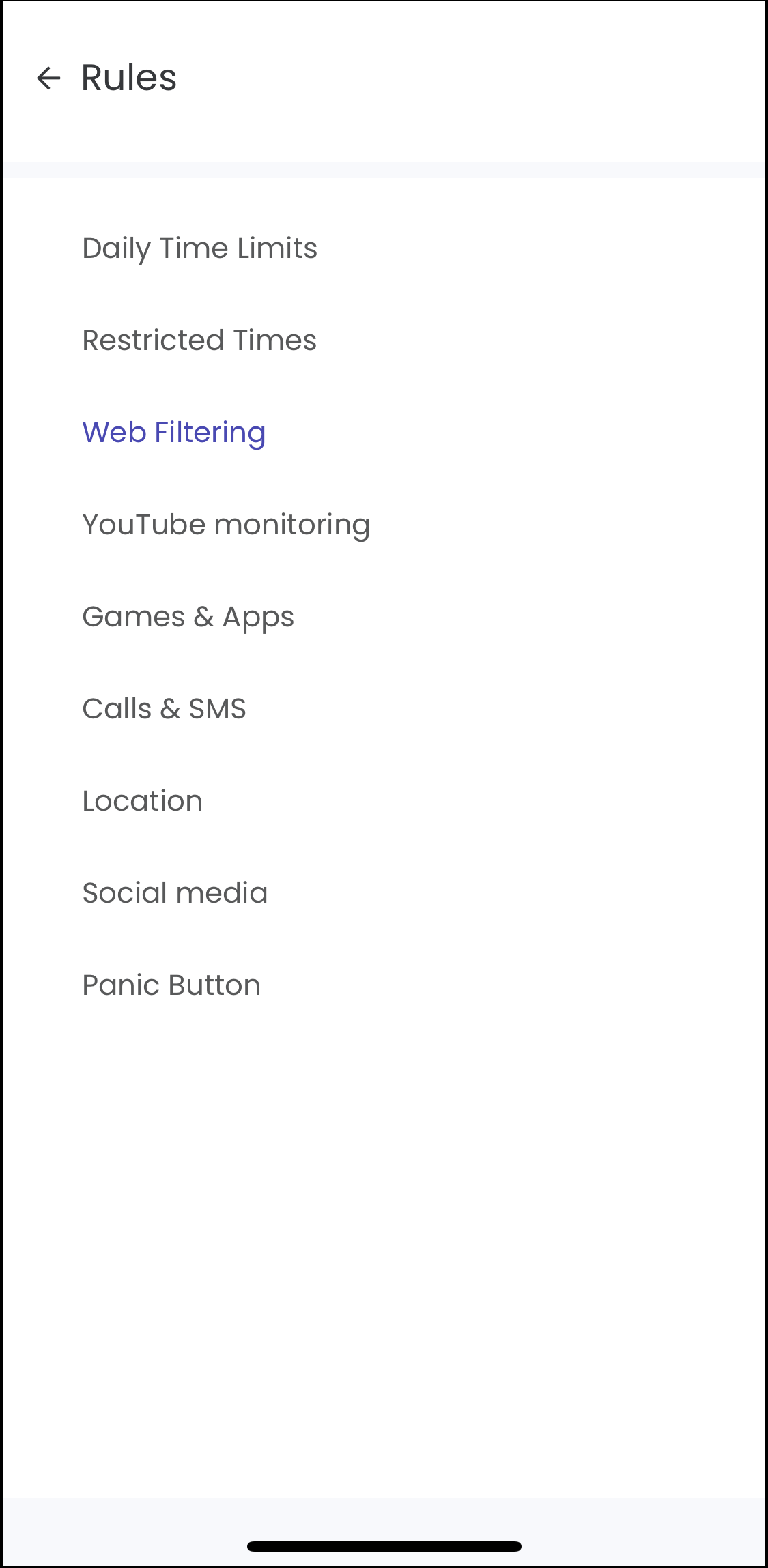In this image, we see the interface of a mobile application, presumably showcasing its settings or parental control features. At the top left corner, the word "Rules" is displayed in black text, accompanied by a left-pointing black arrow. Beneath this, a semi-transparent, light gray rectangular bar spans the width of the screen.

The main section of the screen contains a vertical list of categories. The first item on the list is "Daily Time Limits," followed by "Restricted Times" and "Web Filtering." The "Web Filtering" category stands out as it is highlighted in dark blue text. Continuing down the list, we see additional categories: "YouTube Monitoring," "Games and Apps," "Calls & SMS" (using the ampersand symbol), "Location," "Social Media," and "Panic Button." 

There are notable empty spaces both beneath the list of categories and to the right of each item, indicating either minimal content on this screen or sections awaiting further input.

At the very bottom of the image, another semi-transparent rectangular shape is visible, mimicking the design of the top bar. Centered within this bar, a black horizontal line suggests the presence of a home button, characteristic of many smartphone interfaces.